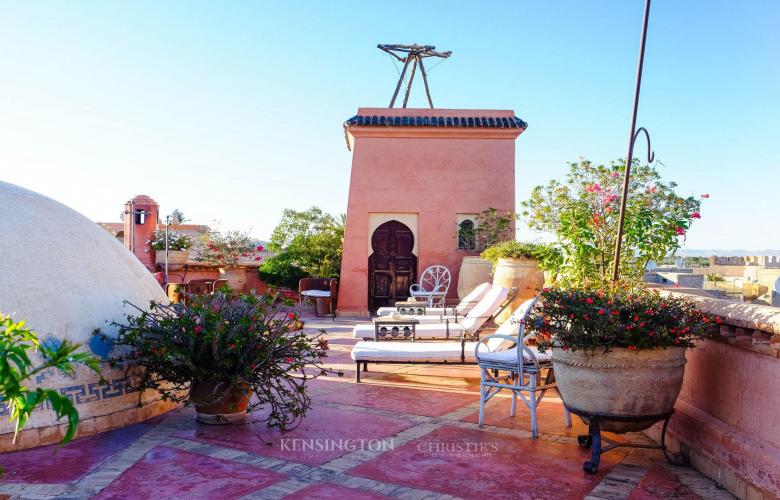This photograph captures a sunlit rooftop patio adorned with distinctive Adobe-style architectural elements, likely situated in a location reminiscent of New Mexico. The ground is covered with large pink tiles articulated by a delicate tan crosshatch pattern. Dominating the left side of the image is a large white stone dome featuring intricate blue tile work at its base. Scattered across the patio are multiple planters containing verdant greenery, adding a touch of nature to the space. 

The seating arrangement includes three white sunbathing chaises aligned horizontally, flanked by two white wire chairs, one at the foot and another at the head. There is also a notable dark wooden door positioned on a prominent rectangular structure at the center of the rooftop. Adjacent to this structure, a tripod-mounted object, perhaps a telescope, draws curiosity.

In the backdrop, the rooftop is bordered by a stone wall on the right, providing a vantage point over a scattering of smaller buildings below. Additionally, there is another circular tower to the left, consistent with the architectural style of the region. The composition subtly hints at an urban setting, possibly New Mexico or a Middle Eastern locale, with "Kensington Christie's" faintly visible at the bottom of the photograph.